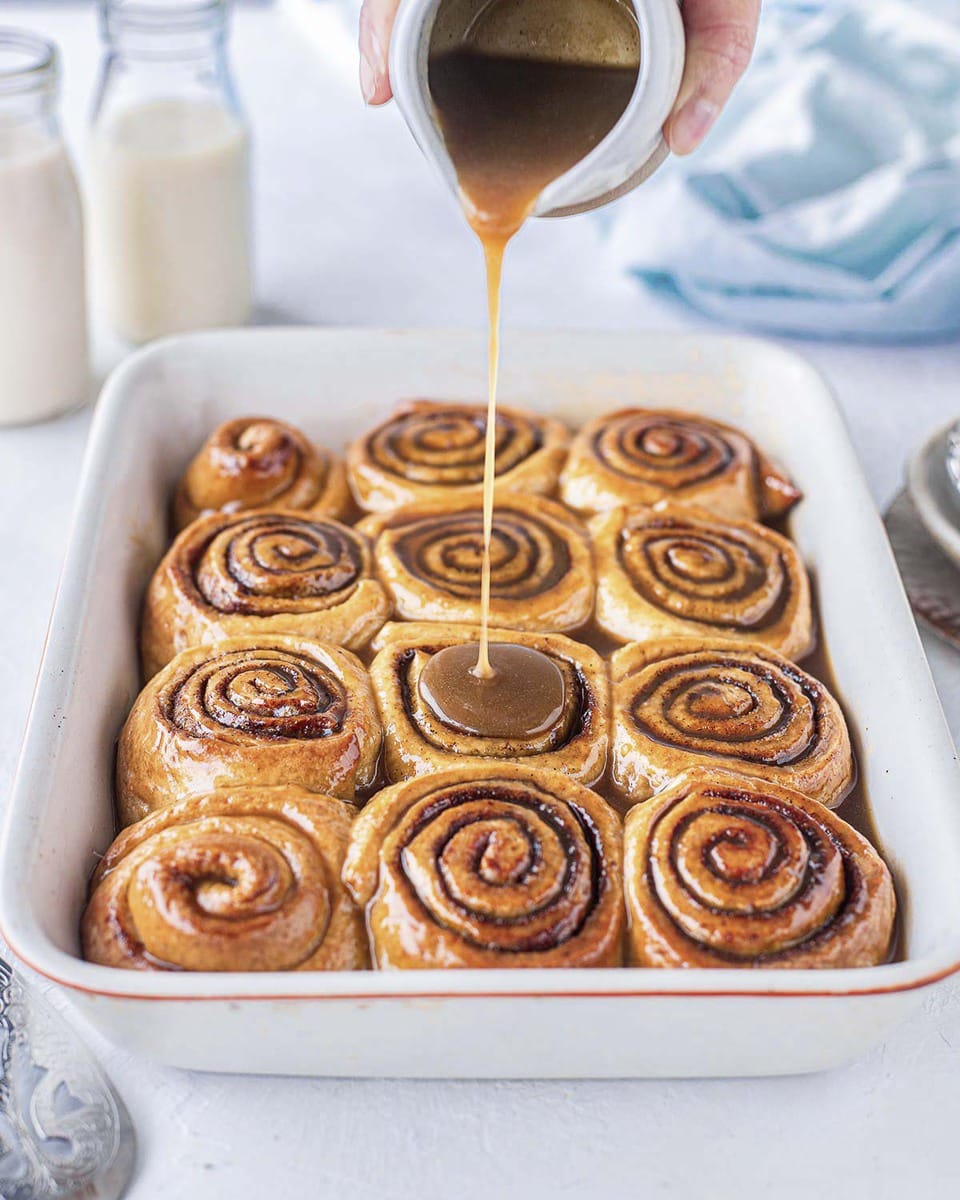The detailed color photograph captures a white enamel baking pan filled with 12 homemade cinnamon rolls arranged in four rows of three. Each roll is a golden tan, intricately spiraled and glistening with dark brown cinnamon in the grooves. At the top center of the image, a hand with Caucasian skin is seen pouring a rich, brown caramel glaze from a miniature white pitcher onto the rolls, adding a glossy sheen. The pan rests on a white surface, and in the background, two clear glass bottles of milk or cream are placed on the left. A wadded-up blue cloth is noticeable in the upper right corner, and the scene is well-lit, showcasing the delectable details of the freshly baked cinnamon rolls and their appetizing presentation.